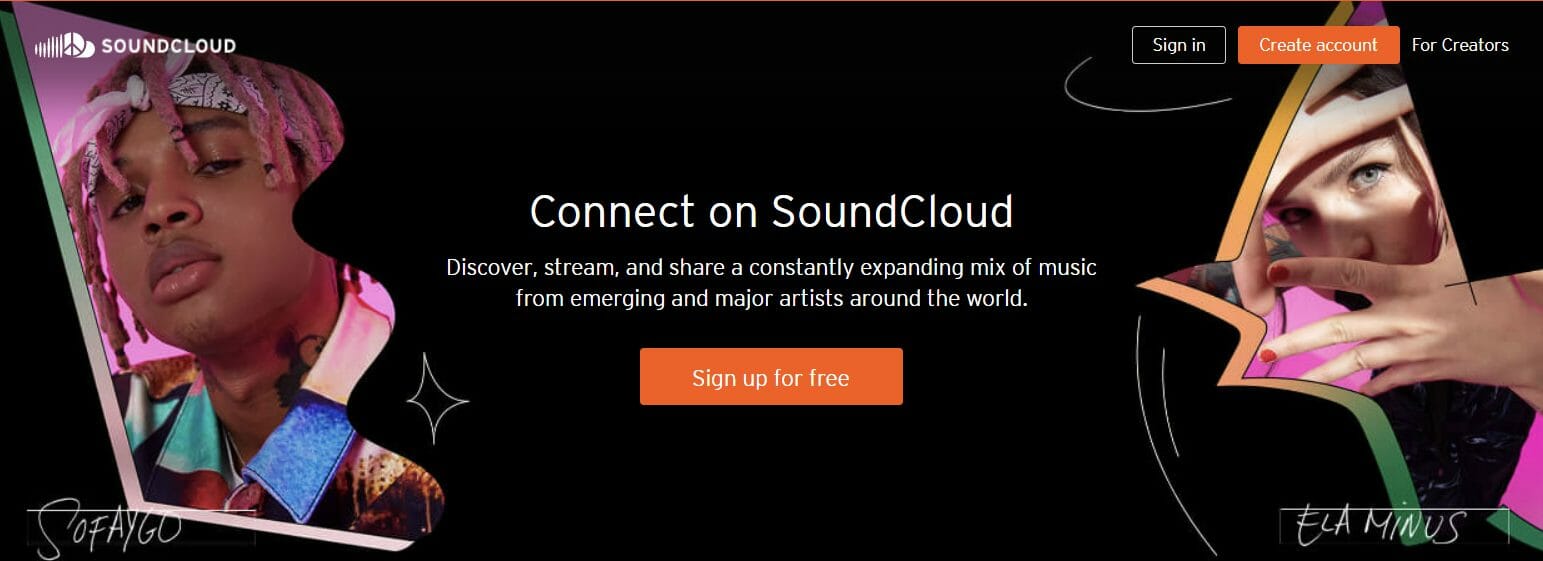In the top left corner of the page, a black rectangle prominently features the white text "SoundCloud." Toward the right side of this header, a button labeled "Create Account" is visible. Meanwhile, on the left side, a photo captures a dark-skinned individual adorned with dreadlocks, and they are sporting a scarf or bandana wrapped around their forehead. Their shirt, which has a collar, is notable for its vibrant gradient transitioning from green to pink to blue.

Centered within the black rectangle, large white letters spell out "Connect on SoundCloud." Beneath this, a tagline reads, "Discover, Stream, and Share a Constantly Expanding Mix of Music from Emerging and Major Artists Around the World," although the exact wording is partially unclear. Following this is a striking red rectangle with white text that reads, "Sign Up for Free."

On the right side of the page, an image of a white woman is superimposed within a star-like shape created by intertwining orange and green ribbons. She strikes a dramatic pose with her right hand resting on her forehead, casting a shadow over her face, revealing only one brightly illuminated eye. Her left hand, adorned with red fingernails, is positioned in front of her face. The woman is also dressed in pink clothing, adding a pop of color to the composition.